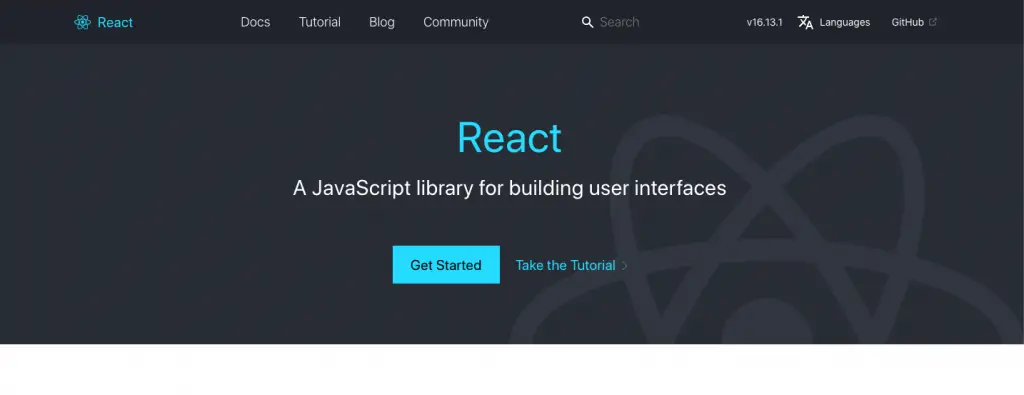The image showcases a webpage with a prominent display of React and its logo in the top left corner. The webpage header includes navigation links for "Docs," "Tutorial," "Blog," and "Community," along with a search bar featuring a magnifying glass icon on its left side. The text indicates the version as 16.1.3.1. The webpage also provides options for selecting languages and links to the GitHub repository. Centrally displayed is the tagline, "React - A JavaScript library for building user interfaces," followed by calls to action such as "Get Started" and "Take the Tutorial." The background is predominantly black, creating a striking contrast with the white and blue text elements used throughout the design.